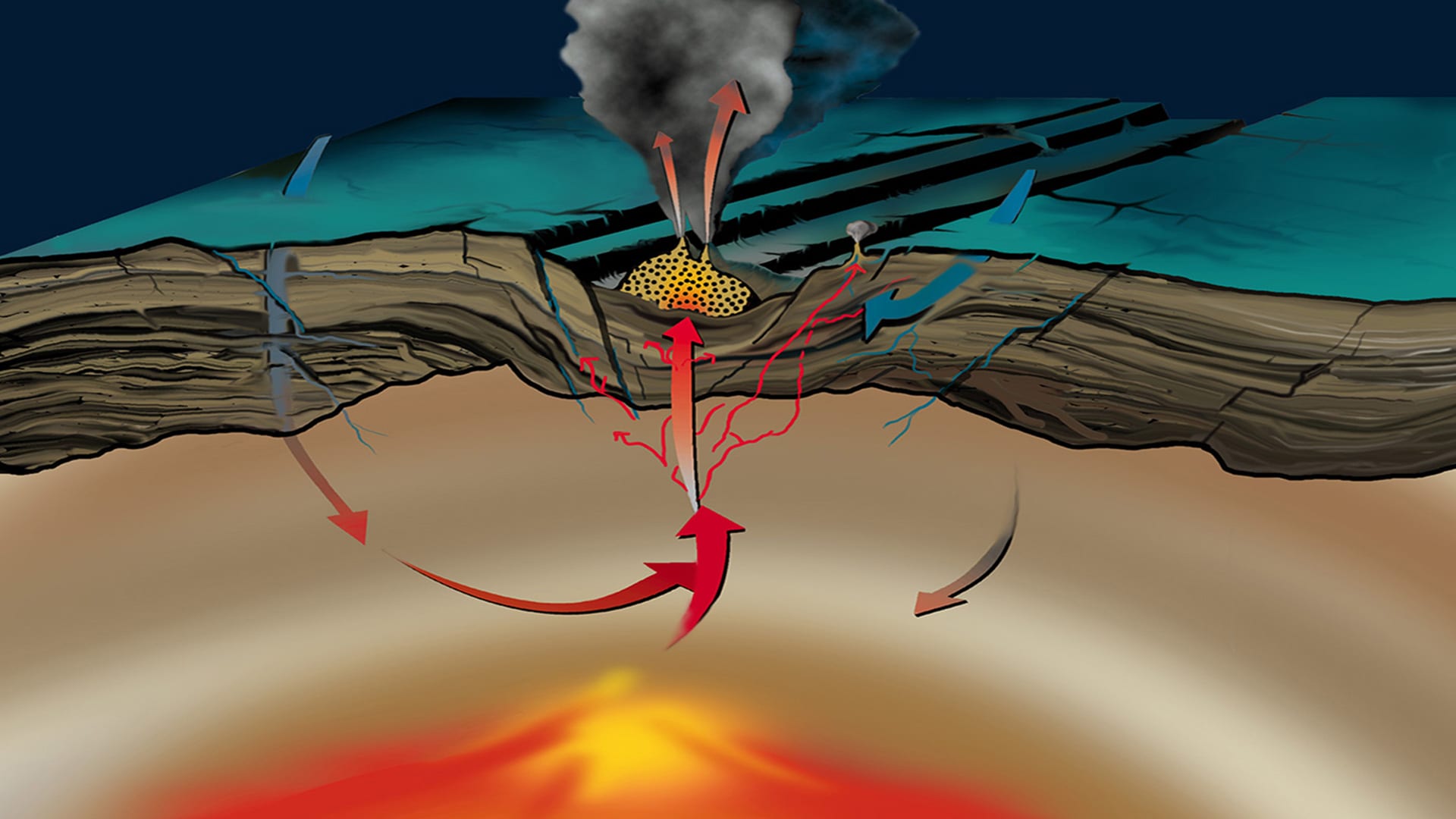The animated image depicts an underground magma flow leading to a volcanic eruption. At the bottom left, there's a blurred depiction of a volcano with red sides and a yellow center. This volcano appears triangular and resides in a brown and tan gradient area, symbolizing the earth's layers. The brown layer, resembling soil or wood, stretches horizontally across the middle, slightly dipping in the center. Above, a dark blue sky transitions to a greenish tint, possibly outlining the land or part of the volcano. 

In the center of the image, there's a pile of yellow circles with black dots, emitting gray smoke. Red and orange arrows point upwards from this pile, indicating the movement of magma. Additional red arrows originate from the very bottom, tracing the path of the lava through the crust, which is shown as layered brown strata. One brown arrow points downwards from this layer towards the volcano. Blue arrows from the sky point downward to the middle section, possibly indicating atmospheric pressure or precipitation.

The upper part of the image features a blue surface, with a trench emerging from the yellow pile, extending upwards and to the right. The entire depiction illustrates the process of magma rising through the earth's crust, leading to a volcanic eruption, characterized by the burst of smoke and upward movement of arrows representing the flow of molten material.